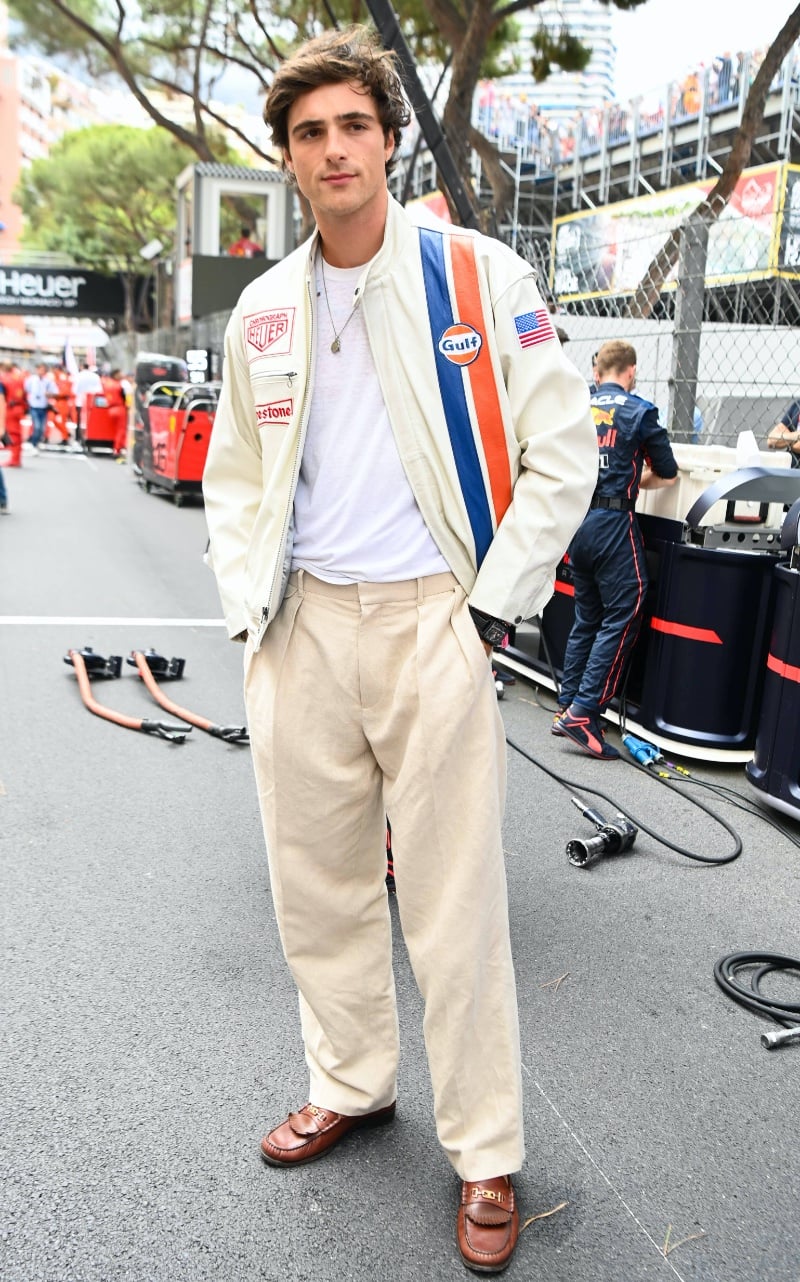In this image, a young Caucasian man, likely in his 20s, stands confidently on a gray asphalt street during what appears to be an outdoor event. He is dressed stylishly in a racing-style beige leather jacket featuring blue and red stripes on the left side. The stripes frame the "Gulf" logo, and on the jacket’s left arm is a patch of the American flag. Underneath, he wears a white shirt and a necklace is visible around his neck. His outfit is completed with light brown khaki pants and dark brown loafers. The man has dark brown, somewhat long hair and appears poised with his hands in his pockets.

In the background, another man with his back turned, dressed in a blue one-piece outfit adorned with yellow and red promotional designs and a black belt, is working on setting up some kind of structure. Surrounding them are various pieces of equipment, including hoses, rusty pipes, and what looks like pneumatic devices. There are blue metal stands on the right side for spectators, a gray chain-link fence, and trees with green leaves. The backdrop includes blurred images of machinery, people, and a distant building under a clear blue sky, alongside a visible gray skyscraper. The scene is bustling with activity, indicative of perhaps a racing event.